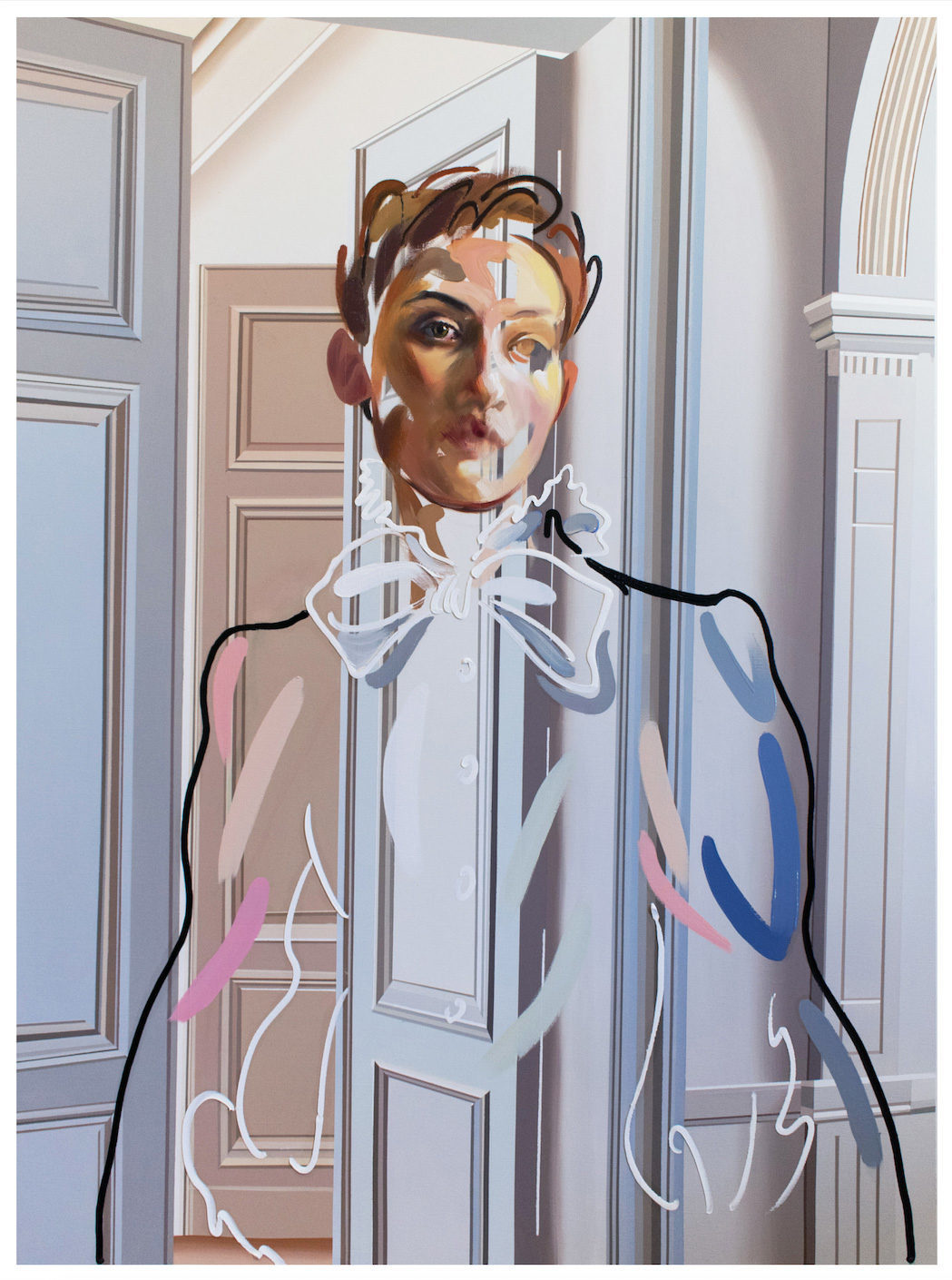This detailed, abstract painting depicts a person in a slightly surreal and unfinished style, positioned centrally in a white, old-style room with partitions, columns, and a series of doors in the background. The figure, who appears to be a woman with light brown, short hair and one detailed brown eye, gazes slightly to the right, as if looking over the viewer's shoulder. Her face is painted in a messy, Impressionist technique, with only partial detail, leaving one eye unfinished. The body of the figure is merely an outline, with sketch-like qualities showcasing folds of a dress suit, a white bow tie, and ruffled collar, all in various light colors like pink, blue, and white. This incomplete depiction makes the figure appear transparent, allowing the viewer to see the detailed room behind her, which adds to the painting's surreal element. The interior features multiple doors, some open and some closed, in paneled frames with intensified edges, contributing to a slightly cartoony effect.